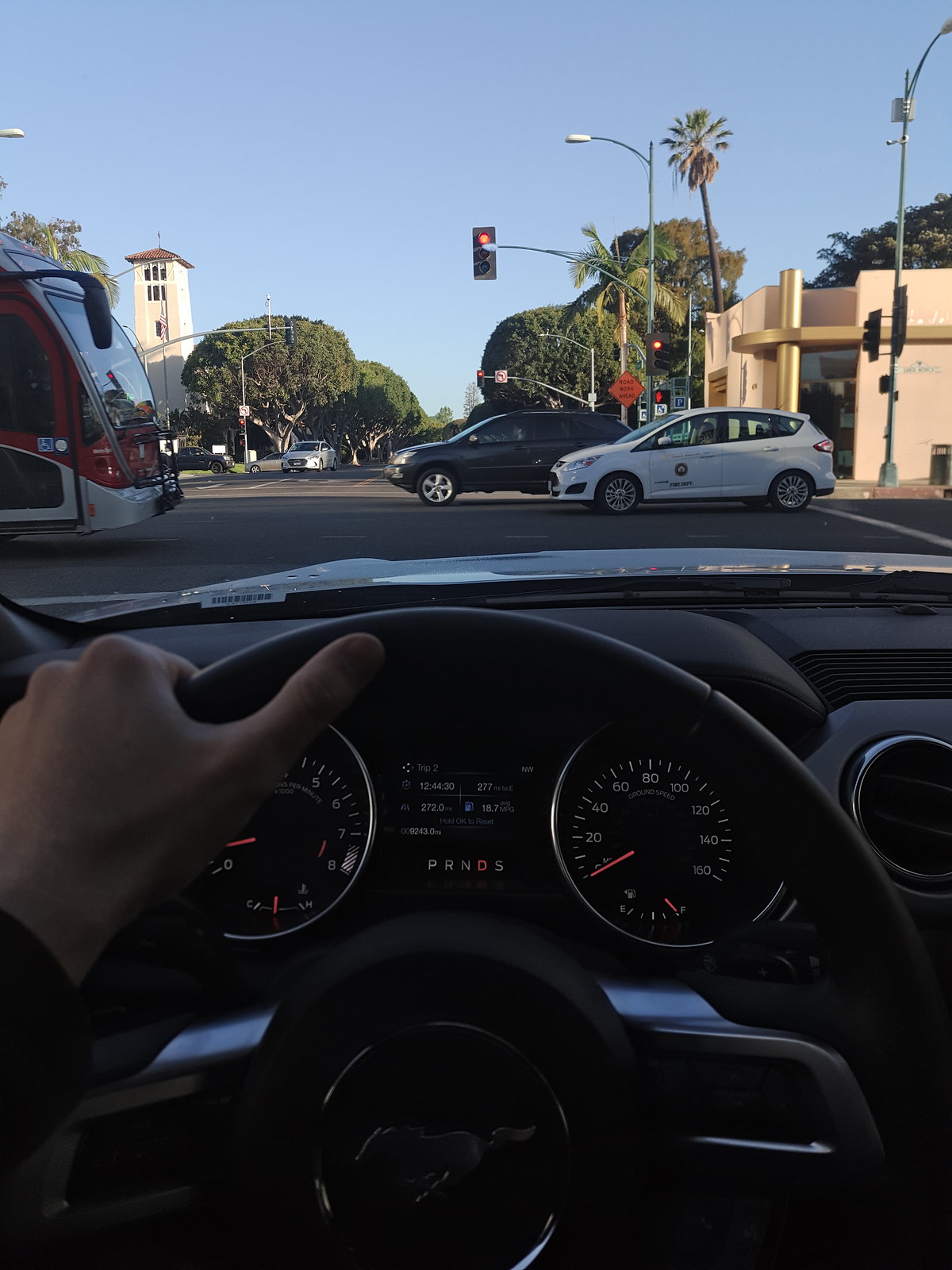The photograph captures the interior view from a Mustang, presenting a scene through the windshield as the car is stopped at a red light at an intersection. The driver's left hand, belonging to a white person, grips the black steering wheel with the iconic Mustang logo prominently displayed in the center. The dashboard, characterized by its black console and white numerical characters, and the speedometer are clearly visible. Beyond the car's hood, the scene reveals a street lined with trees and palm trees on the right. Directly ahead, traffic navigates the intersection, with a red bus moving right and a black minivan and a white two-door car proceeding to the left. The environment features beige and stucco buildings, including a distinct circular structure with an accompanying palm tree, and an American flag perched on a pole, all under a clear blue sky.